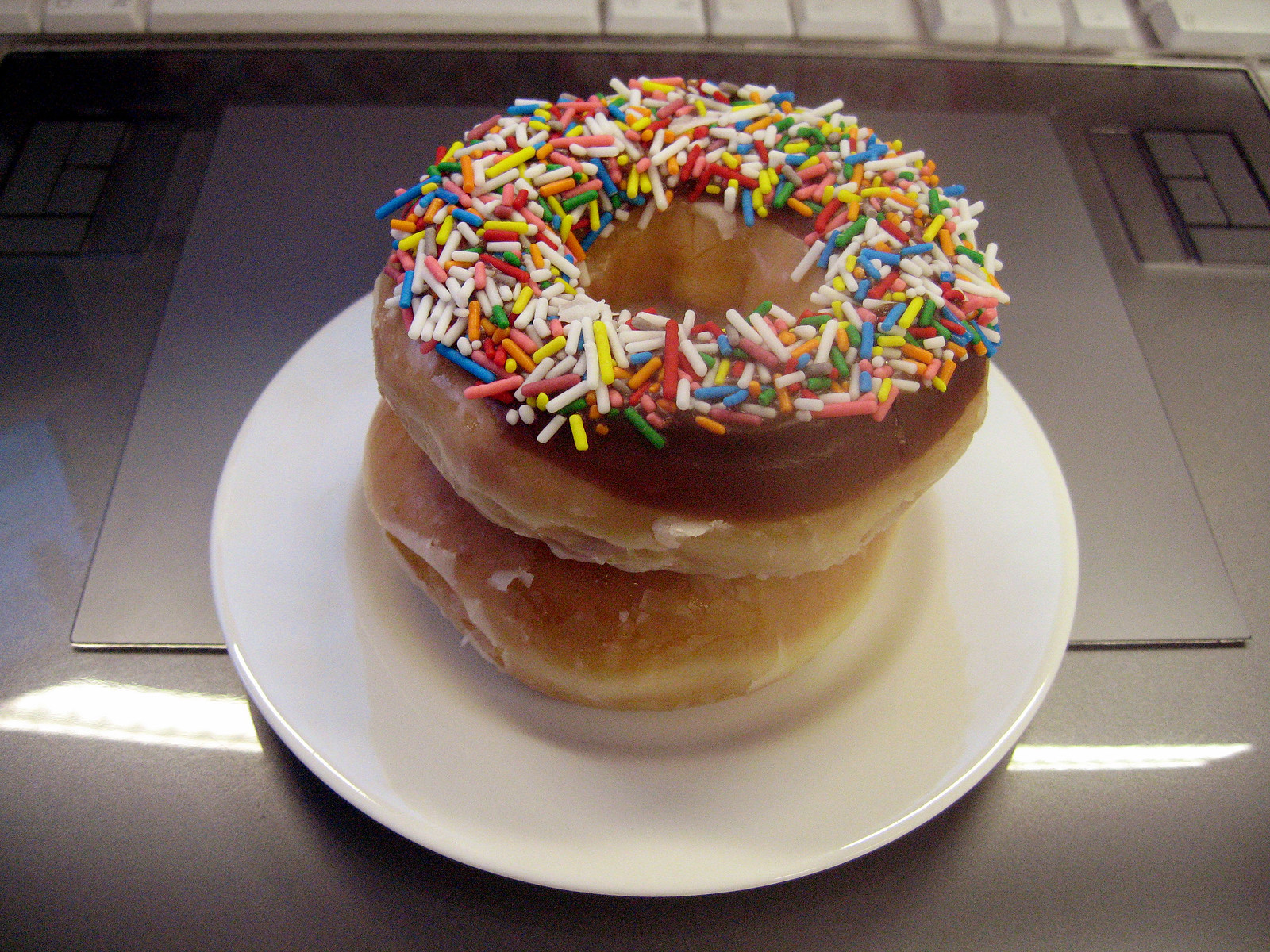The photograph is a close-up, indoor, color image prominently featuring a white ceramic plate placed on a shiny, metallic surface that may be part of a desk or industrial equipment, possibly reflecting ceiling lights. This plate is centered in the image and holds two doughnuts stacked one atop the other. The bottom doughnut is a simple, glazed variety, while the top doughnut is adorned with a thick layer of chocolate glaze and an abundance of multi-colored sprinkles in hues of white, blue, yellow, green, red, and orange. At the very top of the image, there is a partial view of a white computer keyboard. The overall setting suggests an office environment with hints of additional metallic and possible electronic equipment visible in the background, contributing to a slightly varied lighting effect across the image.